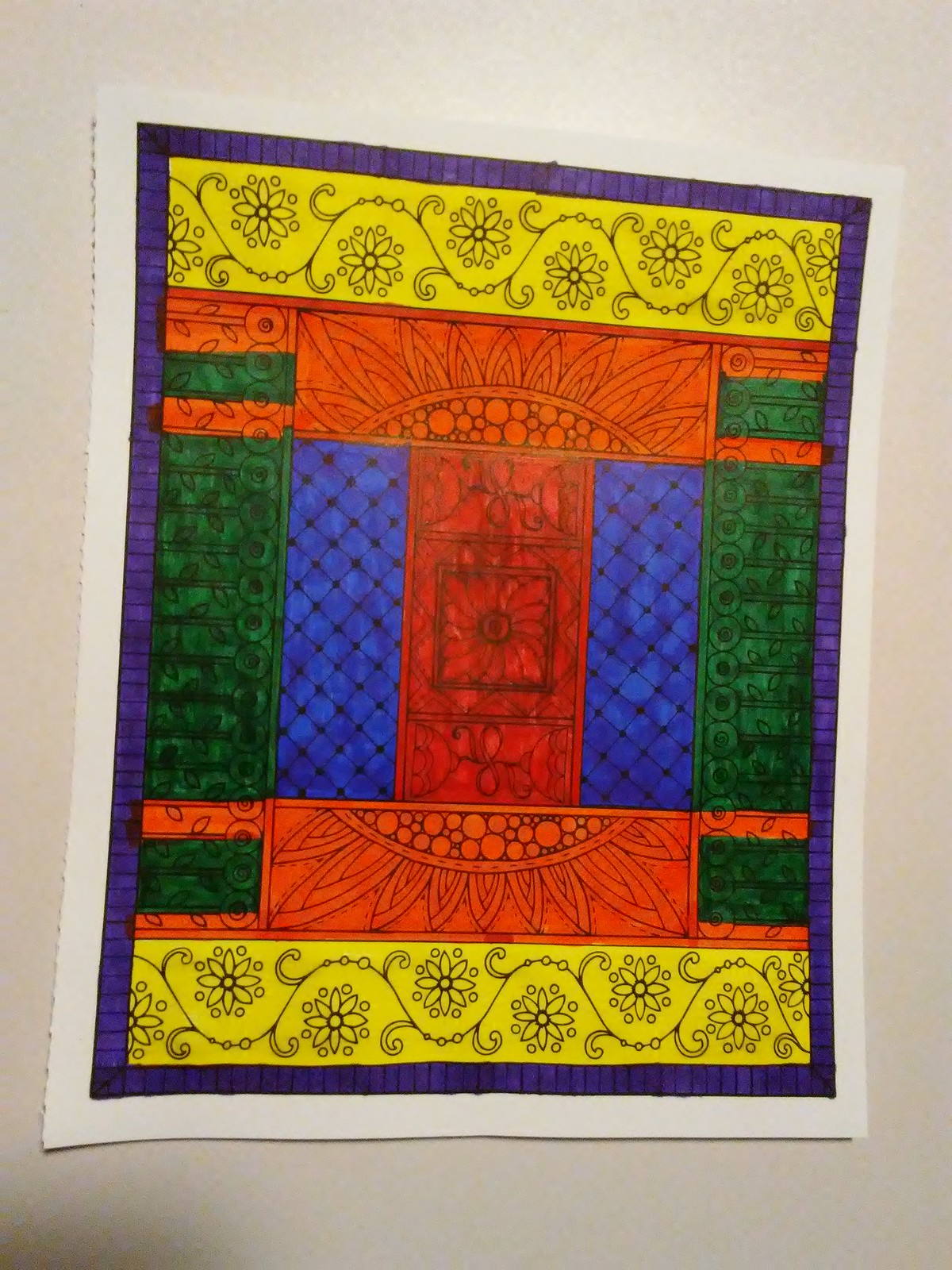This photograph depicts a colorful vertical rectangular piece of paper, which appears slightly off-white and is set against a slightly darker white or off-white background. The paper features intricate colorings that look like they were done with markers on a pre-printed coloring sheet. Surrounding the entire design is a purple border with vertical lines on the top and bottom and horizontal lines on the sides.

At the top and bottom of the paper, there is a yellow section with flower patterns intertwined with vines that create a mountain-like shape. These flowers are arranged alternately above and below the vines and resemble either sunflowers or daisies, with large petals and uncolored circular centers.

Beneath the top yellow section is an orange area that contains flower-like petals. On the left and right edges of this orange section, there is some green.

Next, there is a larger green section on the left and right edges, forming vertical rectangles that frame the subsequent central designs. Inside this green frame, there is a dark blue area with black circles forming diamond shapes.

At the center of the image is a reddish-orange rectangle with a black square containing a circular center. Below this reddish-orange rectangle is another orange section with a semicircular design outlined in black, filled with varying sizes of orange dots, and petals extending from the semicircle that point downward.

Repeating the top yellow section, the bottom of the image also includes yellow flowers with vines creating a symmetrical balance to the overall design. A slight shadow can be seen on the bottom portion of the page, adding depth to the image.